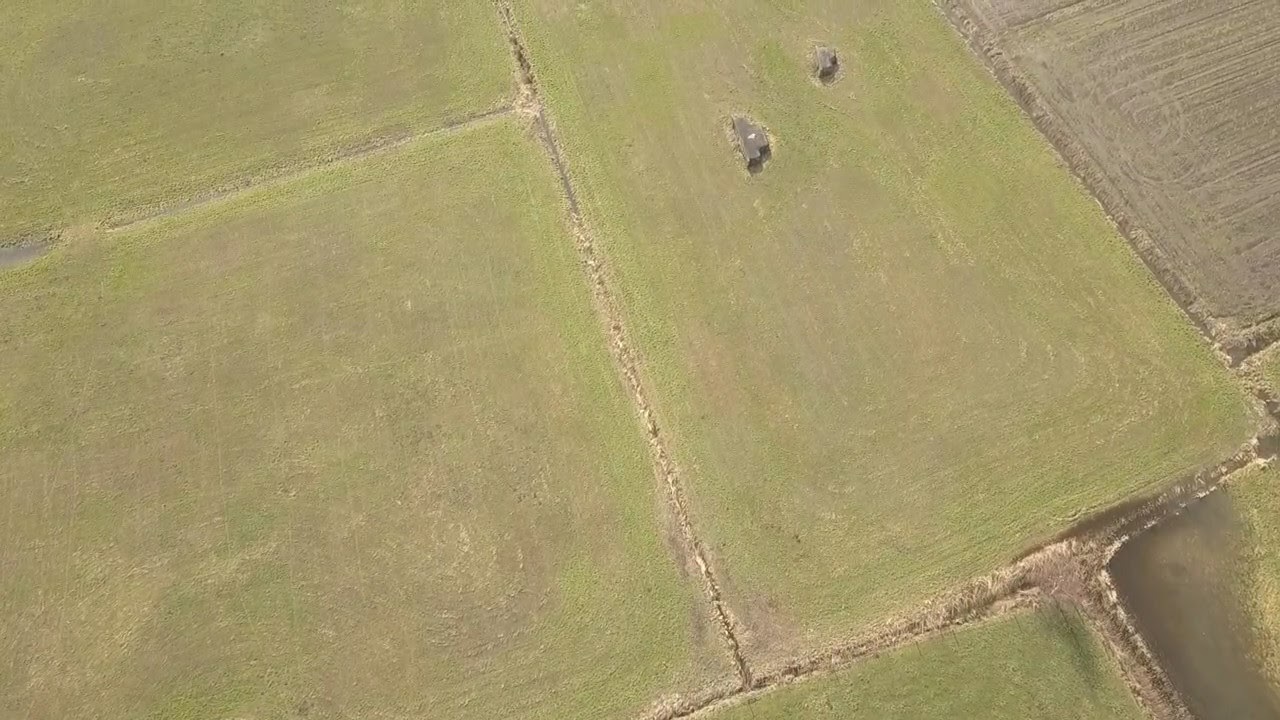This detailed aerial view, captured by a drone, showcases a patchwork of rectangular sections of farmland. The photograph, likely taken in the fall or winter, reveals seven fields, although five extend beyond the frame. These fields have clear borders, suggesting property lines. Most sections exhibit various hues of yellowish-green grass, typical of the season. The central field stands out with two large boulders, adding a unique landmark within the otherwise uniform rows. On the right side of the image, one field shows signs of recent tilling with visible lines in the brown soil, indicating preparation for planting. Similarly, on the bottom right, another field has brown soil, possibly flooded, hinting at water accumulation. This geometric arrangement of fields, with a mixture of greenery and bare soil, gives a comprehensive overview of the agricultural landscape from a high perspective.